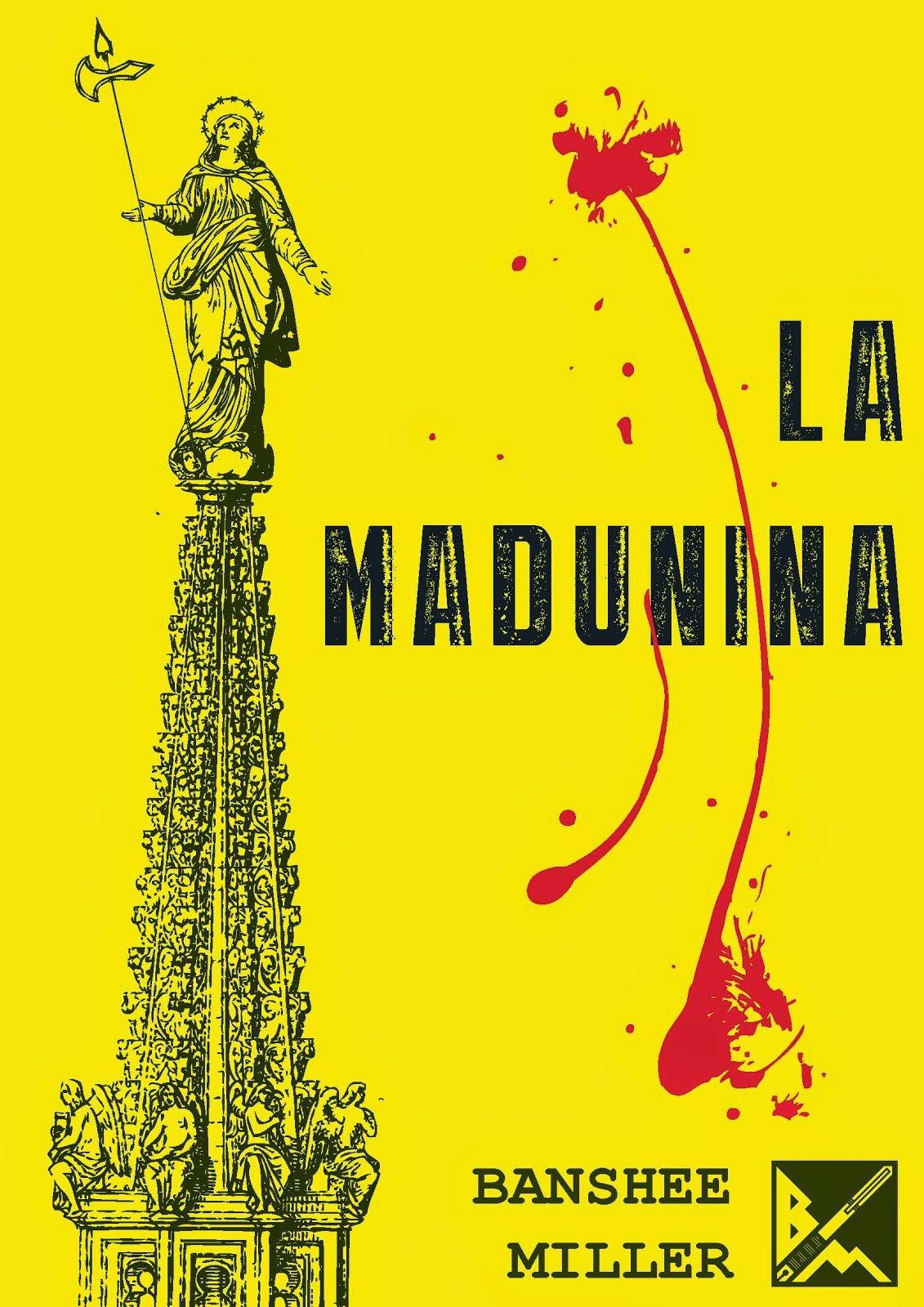The poster features a vibrant yellow background with a prominent black spire of an intricate, old building on the left side. This ornate spire is adorned with four angels sculpted at its base and an elaborate column that culminates in a small platform. Atop this platform stands the statue of a saint, possibly Mary, holding what looks like an axe in one hand and wearing a halo. To the right of the spire, bold black letters spell out "LA MADUNINA," with red splatters resembling blood crossing through the letters. In the lower right-hand corner, the text "Banshee Miller" appears in black letters, accompanied by a logo or emblem featuring a black and white box with an object, possibly a sword, running through its center. The visual elements and striking colors suggest an advertisement or promotional material.